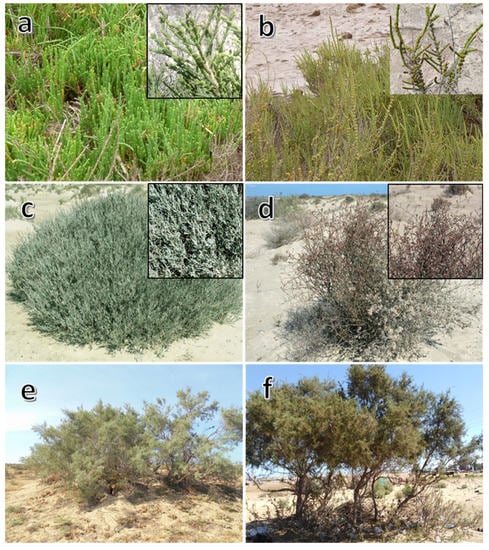This image is a composite of six labeled photos (A–F) showcasing various types of desert vegetation. Arranged in a grid with A at the top right, B to its left, C in the middle right, D in the middle left, E in the bottom right, and F in the bottom left, each small photo captures different plant life. 

Photo A features green grass, vibrant in color. Photo B shows longer grass, distinctly light green. Photo C depicts a patchy, pine green area of short grass in a somewhat circular formation. Photo D presents a light brown plant, appearing dead or dried out. Photo E highlights a light green bush, low to the ground. Lastly, Photo F displays a green tree with brown branches extending outward, looking more vibrant than its counterparts.